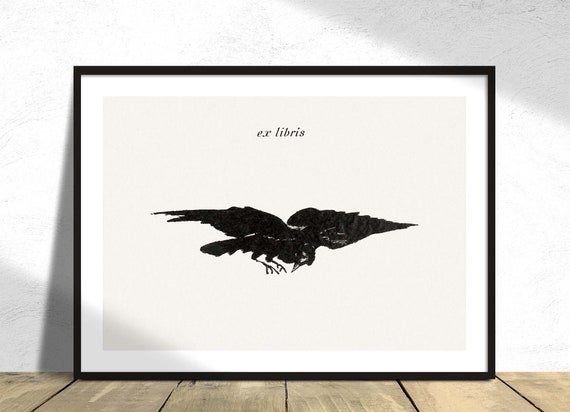This horizontally aligned rectangular image showcases a black-framed picture propped against a textured white wall with light gray accents. The floor beneath, made of medium brown vertical wood slats, partially visible, resembles a plank floor or wooden table. The picture frame is thin, black, and houses a white mat leading into a large, beige background. The top of the picture bears the text "Ex Libris" in smallish letters. Central to the image is a black bird with wings outstretched, viewed from a slightly top-down angle, with its head tilted downward and feet visible beneath it. The depiction of the bird exhibits shaded details primarily in black, creating a striking contrast against the lighter background.